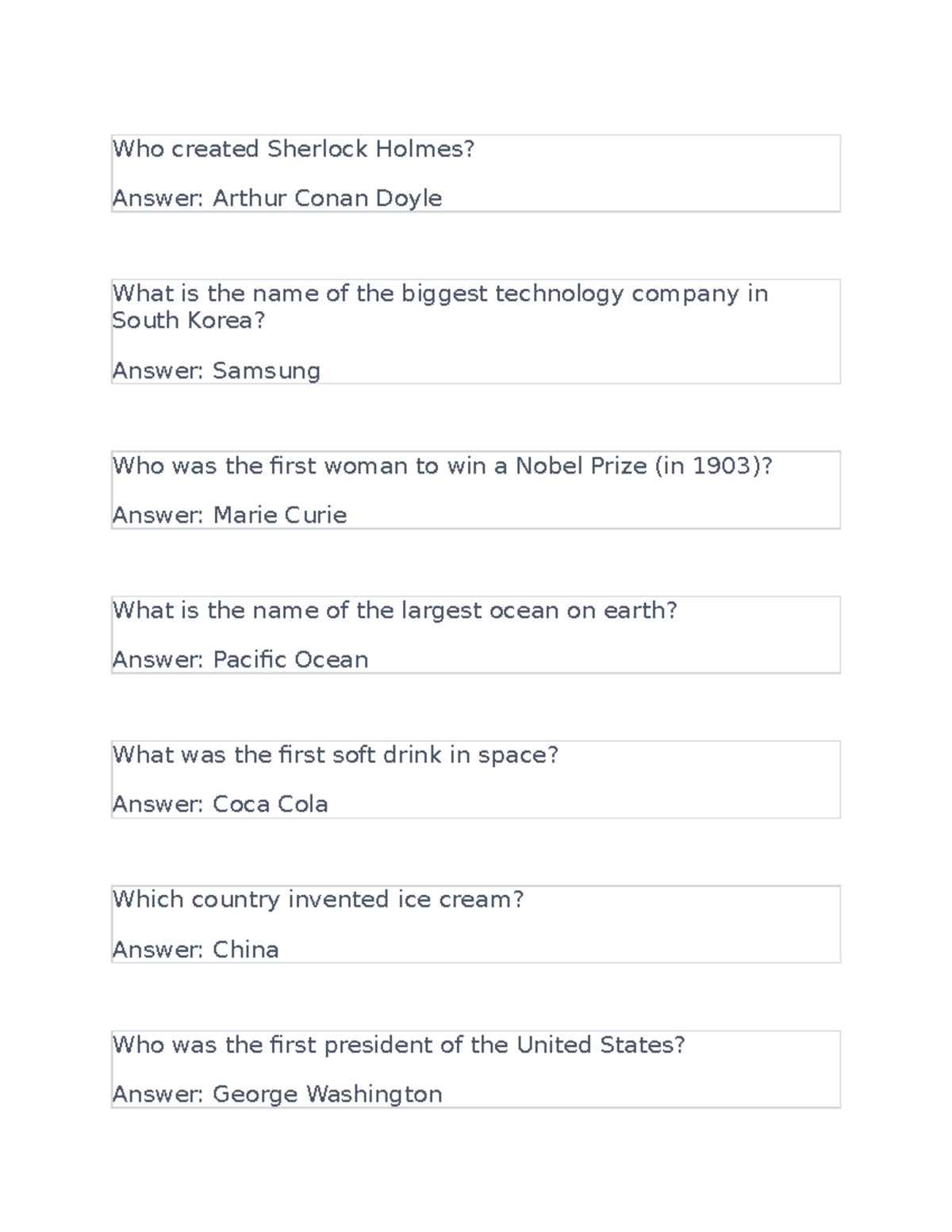In the image, a series of trivia questions and their corresponding answers are displayed in black text against a white background. The questions and answers are arranged vertically, each encapsulated in a thin, gray, rectangular border for clarity. At the top, the first question reads, "Who created Sherlock Holmes?" with the answer, "Arthur Conan Doyle," immediately beneath it. Following this, the next question asks, "What is the name of the biggest technology company in South Korea?" with "Samsung" provided as the answer. 

Continuing down the list, another question inquires, "Who was the first woman to win a Nobel Prize in 1903?" with "Marie Curie" noted as the answer. The subsequent question poses, "What is the name of the largest ocean on Earth?" answered by "the Pacific Ocean." Moving further, the trivia states, "What was the first soft drink in space?" with "Coca-Cola" as the response. 

The penultimate question is, "Which country invented ice cream?" with the answer, "China." Lastly, the query, "Who was the first President of the United States?" is answered by "George Washington." Each question and its respective answer are distinctively separated by their thin, gray-bordered rectangles, providing an organized and structured layout. This comprehensive image encapsulates a set of intriguing facts, neatly presented from top to bottom.